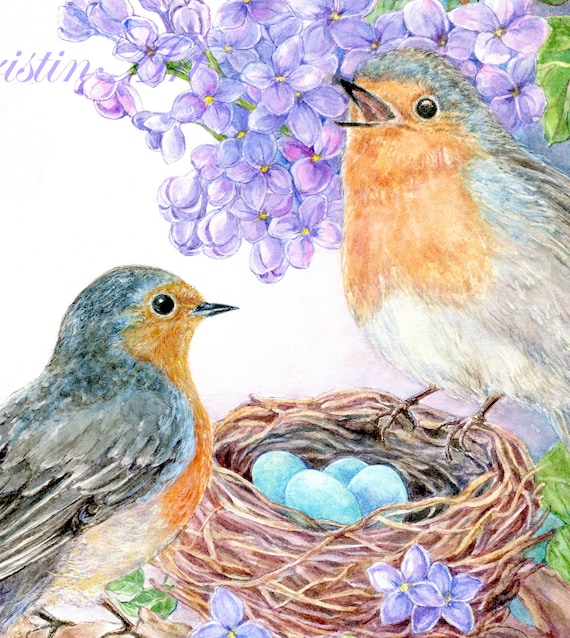This detailed pastel or watercolor drawing depicts a lively spring scene featuring two robins perched adjacent to their neatly woven nest on a tree branch. The larger robin, characterized by its orange belly, grayish-bluish feathers, and a pointed black beak, appears to be singing with its mouth open. The smaller robin, similarly feathered, sits by the nest which cradles several turquoise, robin-sized eggs. The backdrop is predominantly white, accentuated by the vibrant lilac and pink blossoms along with hints of green leaves, suggesting a blooming spring. The meticulous details in the birds, their nest, and the flowers exhibit the artist's skill, creating an image reminiscent of an invitation cover.